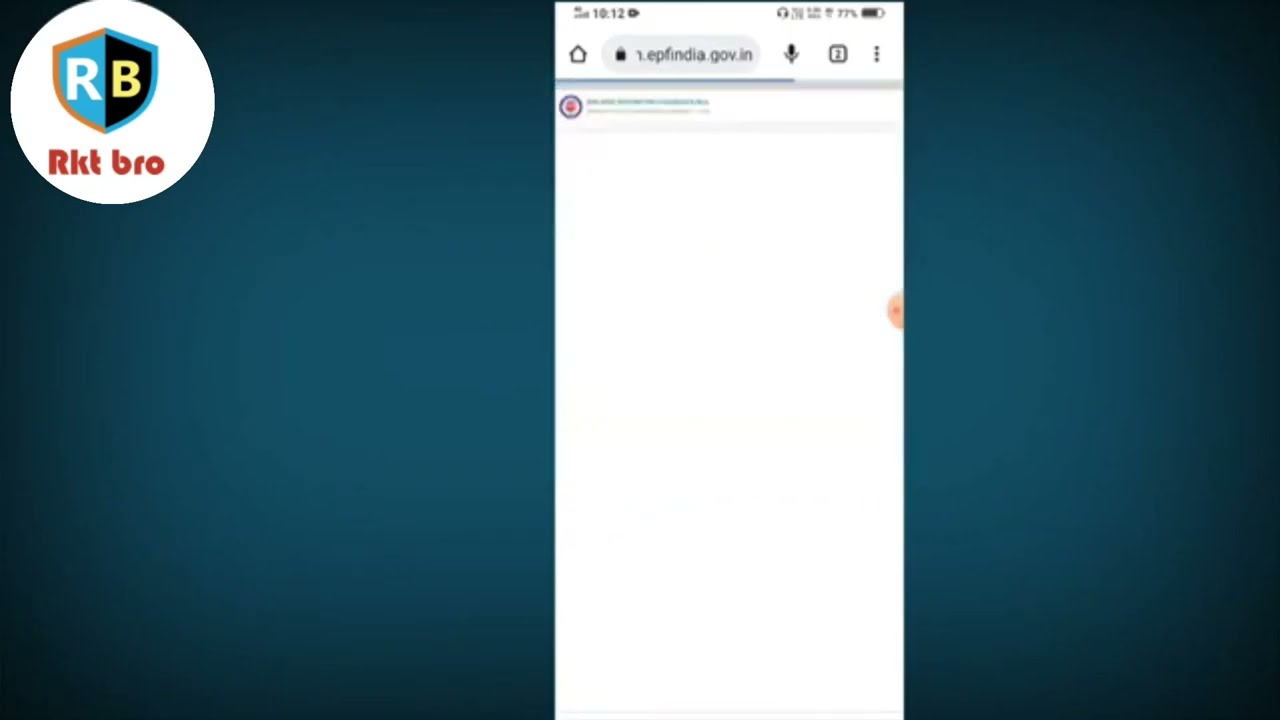The image appears to be a screenshot, possibly from a phone screen, featuring a web browser. The backdrop is a dark bluish-green color with darker edges. In the upper left corner, there's a white circle enclosing a shield emblem split into blue and black halves with the letters "R" and "B" inside, the "R" in white on the blue half and the "B" in yellow on the black half, accompanied by red text below the circle reading "RKT BRO." The center of the image showcases a vertical white rectangle, resembling a browser screen, flanked by the dark bluish-green background. Across the top of the screen, there's a gray URL bar displaying "epfindia.gov.in," along with various icons including a home symbol, a microphone, and indicators for battery life (77%), signal strength, and the time (10:12). Below the URL bar is predominantly blank, suggesting the browser page hasn't fully loaded or navigated to a website yet.